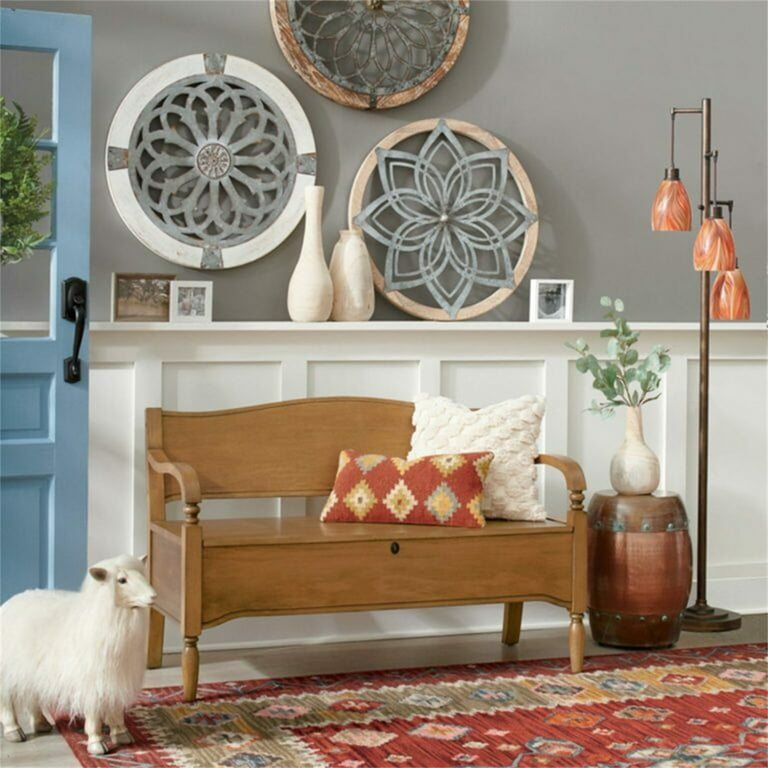The image showcases a pristinely maintained room decorated in a Pennsylvania Dutch style. The walls are gray on the upper half and white on the bottom half, featuring three circular spirograph-like artworks in shades of gray and white. An ornate oriental carpet with diamond patterns covers the floor. Positioned in the entryway is a wooden bench with two decorative pillows, one red and one white. To the right of the bench, an end table fashioned from a small whiskey keg barrel holds a white vase with foliage. A dark bronze floor lamp with multiple orange lampshades is situated nearby. To the left of the bench, a stuffed sheep sits on the floor in front of an open blue door, which boasts a wrought iron black handle and a green wreath. Above the bench, a wooden ledge displays three framed photographs and two white vases. The overall scene is one of immaculate and thoughtful decor, blending traditional elements with subtle modern touches.